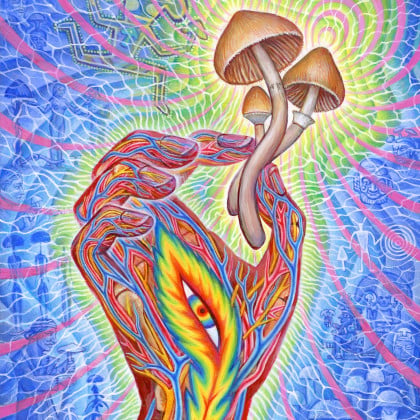This psychedelic image, whether painted or computer-animated, presents a captivating visual feast. At its center is a left hand, slightly closed and extending upward from the bottom of the frame, where the fingertips face to the right. The hand sports a vibrant color palette: red on the outside with blue and yellow veins running through it. An intricate, multicolored eye—featuring black, red, yellow, green, and blue hues—is embedded in the palm, framed by feather-like designs. The hand holds three mushrooms, each with white stems and light to dark brown caps; a larger one reaches toward the top, flanked by two smaller ones. The mushrooms' placement adds depth to the scene, emphasizing the hand's grip on them. A yellowish-greenish glow surrounds the hand, enhancing its otherworldly appearance. The blue background is rich with elements such as people standing, chatting, and running, as well as more fantastical elements like aliens and skulls. Red swirly lines traverse the background, adding to the overall tie-dye, psychedelic effect. The image combines vivid colors and hidden details to evoke a sense of surrealism and perhaps hints at themes of mind-expansion.